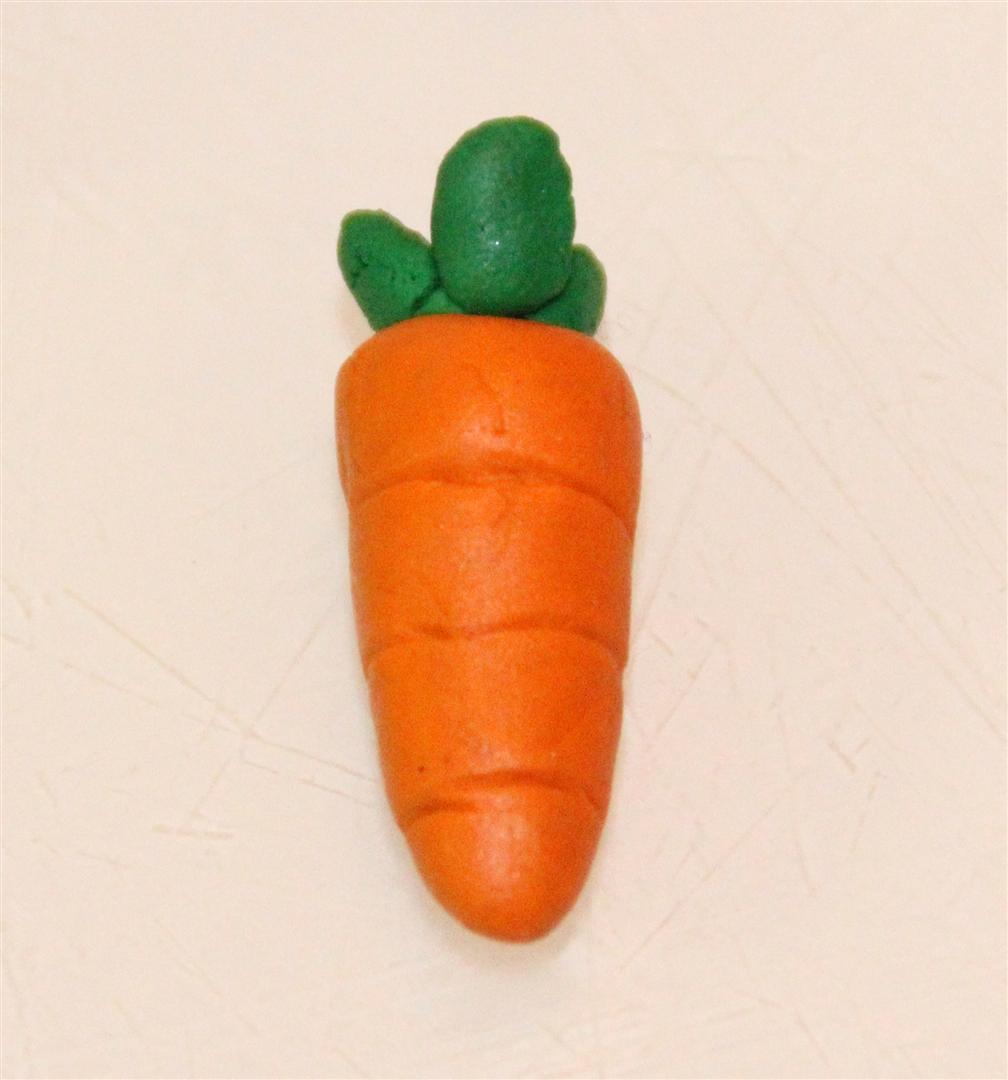The image features a realistic-looking, miniature carrot decoration set against a white background, which appears to be a close-up shot of the surface of a cake. The carrot itself is short and stumpy, with an orange body and three green leaves sprouting from the top. There are subtle indications that the "carrot" is actually made from edible materials like candy frosting or fondant. The background, likely a layer of white frosting with pale cream lines, exhibits a textured appearance reminiscent of an old Formica surface, hinting at a slightly vintage aesthetic. The photograph is taken from an overhead perspective, centering the carrot in the frame.